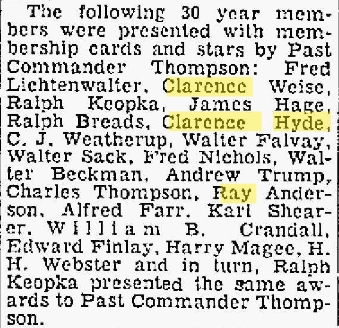The image is a small, square-shaped cutout from a newspaper, featuring black text on a white background, bordered by thin lines on the left and right sides. It announces that the following 30-year members were presented with membership cards and stars by past Commander Thompson: Fred Lichtenwalter, Clarence Weiss (highlighted in yellow), Ralph Koepka, James Haig, Ralph Breeds, Clarence Hyde (highlighted in yellow), C.J. Witherup, Walter Falvey, Walter Sack, Fred Nichols, Walter Beckman, Andrew Trump, Charles Thompson, Ray Anderson (highlighted in yellow), Alfred Farr, Carl Scheer, William B. Crandall, Edward Finley, Harry McGee, and H.H. Webster. Additionally, it notes that Ralph Koepka, in turn, presented the same awards to past Commander Thompson.